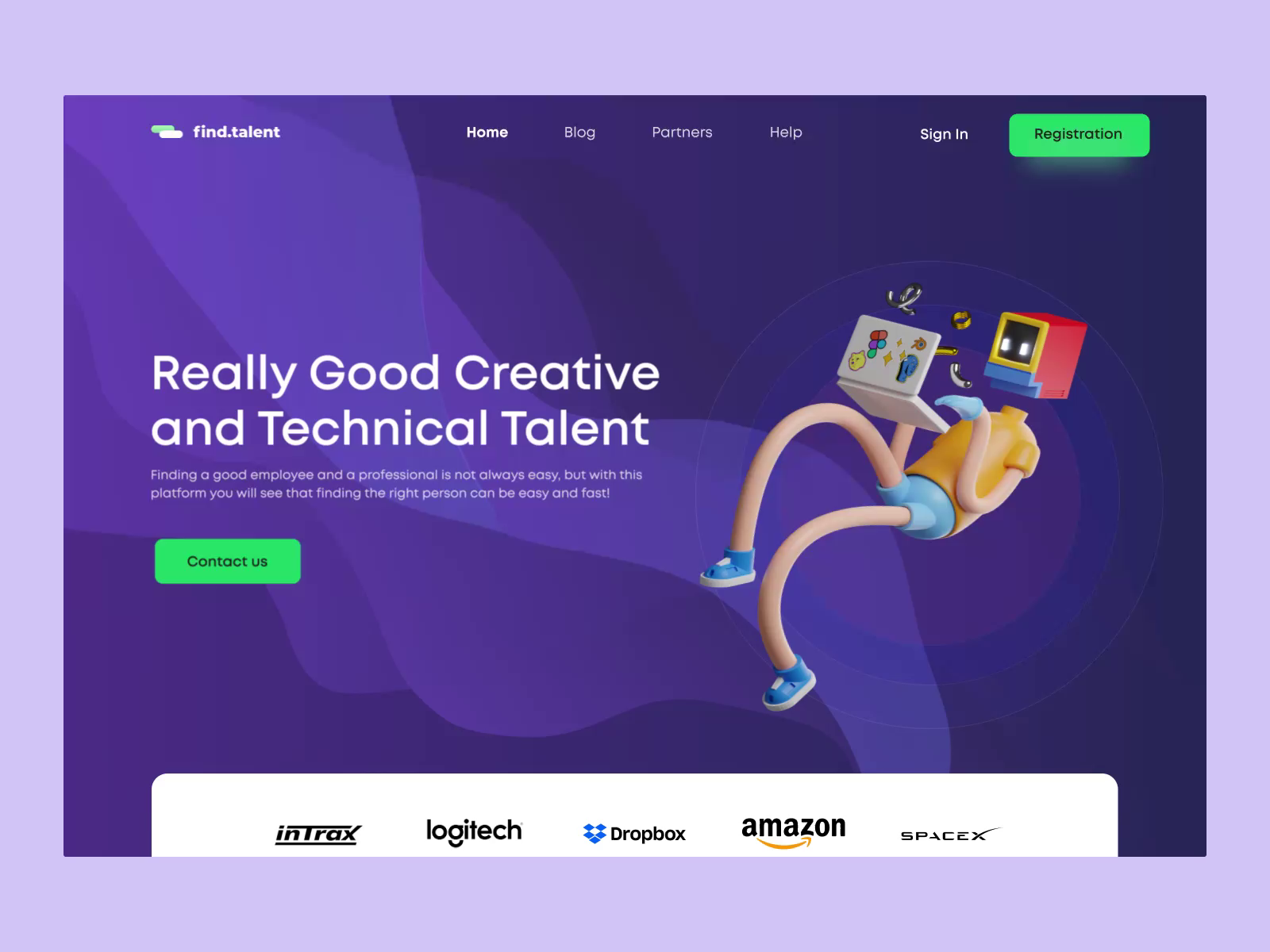The image features a website interface primarily designed to help users find talent. The website name "Find.Talent" is prominently displayed in the top left corner. The navigation bar includes options such as Home, Blog, Partners, Help, with Sign-In and a bright green Registration button located on the right-hand side.

The overall color scheme of the webpage is a gradient of purple and blue, resembling a waveform. The central visual element is an illustration of a robot-human hybrid. This figure has human-like limbs clad in shorts, an orange t-shirt, and blue shoes, but its head is distinctly robotic. The character is reclined backward while typing on a laptop, positioned towards the middle-right of the image.

On the middle-left of the image, a bold white text declares, "Really good creative and technical talent." Below this, in smaller white text, the caption explains, "Finding a good employee and a professional is not always easy, but with this platform you will see that finding the right person can be easy and fast." Underneath this text, there is another green box labeled "Contact Us."

At the bottom of the webpage, separated by a white box, are the logos of well-known companies: Intrax, Logitech, Dropbox, Amazon, and SpaceX, highlighting partnerships or endorsements.